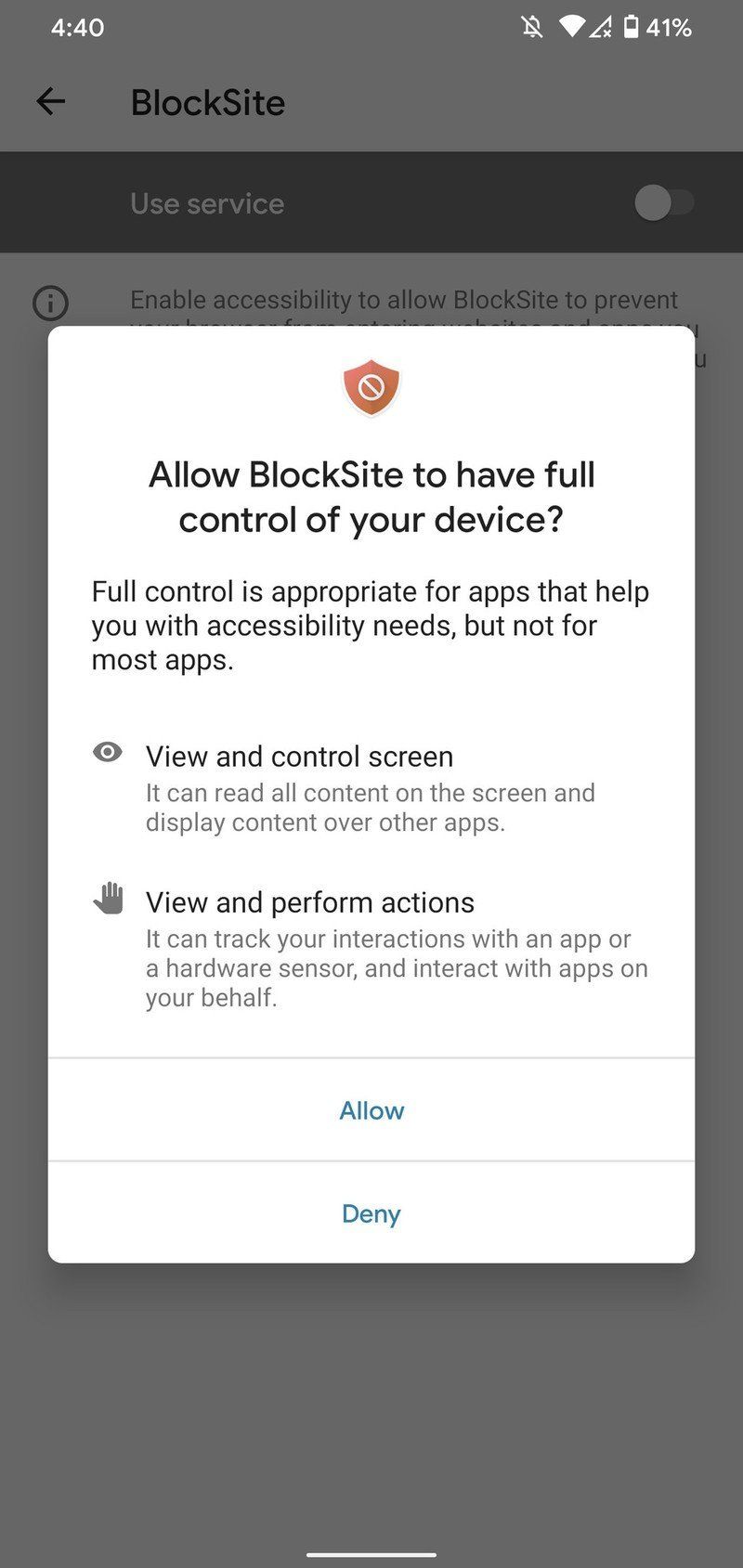The image depicts a "Device Control" notification box that is overlaying a grayed-out background screen. The notification appears to belong to an app termed "Block Site," requesting extensive permissions to operate on the device.

At the top of the gray background screen, "Block Site" is written in bold black text. Below this, aligned to the left, there's a back arrow positioned next to a toggle button labeled "Use service," currently set to "Off." Adjacent to this setup, an icon in the shape of an eye accompanied by the message "Enable accessibility to block" is present.

The subsequent text states, "Allow Block Site to prevent," followed by what seems to be truncated information. Directly beneath this, the message continues to indicate: "Allow Block Site to have full control of your device. Full control is appropriate for apps that help with accessibility needs but not for most apps."

The notification box displayed over this background conveys the primary message: "View and control the screen." It elaborates that the app "can read all content on the screen and display content over other apps." This statement is followed by a separate point: "View and perform actions," clarifying that the app "can track your interactions with an app or a hardware sensor and interact with apps on your behalf."

Finally, at the bottom of the notification box, two options are presented: "Allow" and "Deny." A horizontal white navigation bar overlays the bottom of the dark gray screen, providing contrast to the gray background.

This comprehensive screenshot highlights the significant level of access that the "Block Site" app requests, which may be disproportionate for apps that do not cater specifically to accessibility needs.